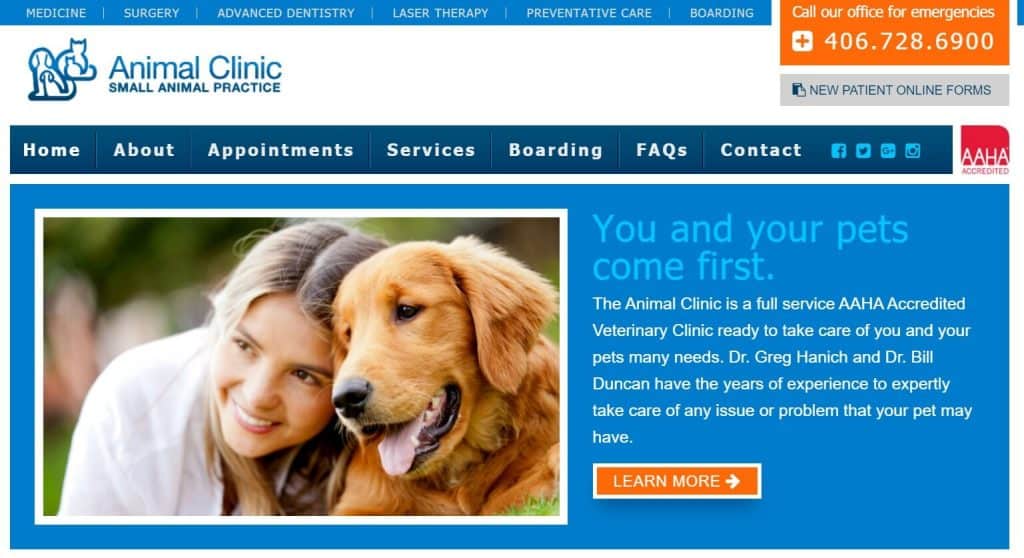A cropped screenshot of an animal hospital's website showcases a coherent and informative layout. 

At the top left, the logo for "Animal Clinic Small Animal Practice" stands clearly. Spanning the top, a blue header offers various categories including "Medicine," "Surgery," "Advanced Dentistry," "Laser Therapy," "Preventative Care," and "Boarding." 

On the top right, a prominent orange box with a plus icon and a telephone number urges visitors to "Call Our Office for Emergencies." Below this, a grey button is labeled "New Patient Online Forms."

A large blue navigation bar stretches horizontally across the middle of the screenshot, listing options such as "Home," "About," "Appointments," "Services," "Boarding," "FAQ," and "Contact." To the right of this bar, small square social media icons are displayed. At the far right, the AAHA (American Animal Hospital Association) logo is visible.

Further down, another large blue box is present. Dominating the left side is a large square photo of a child and a dog, symbolizing the clinic's family-friendly approach. On the right, the phrase "You and your pets come first" is boldly printed in blue font. Below this, a brief description of the clinic is provided. Concluding this section, an orange button encourages visitors to "Learn More."